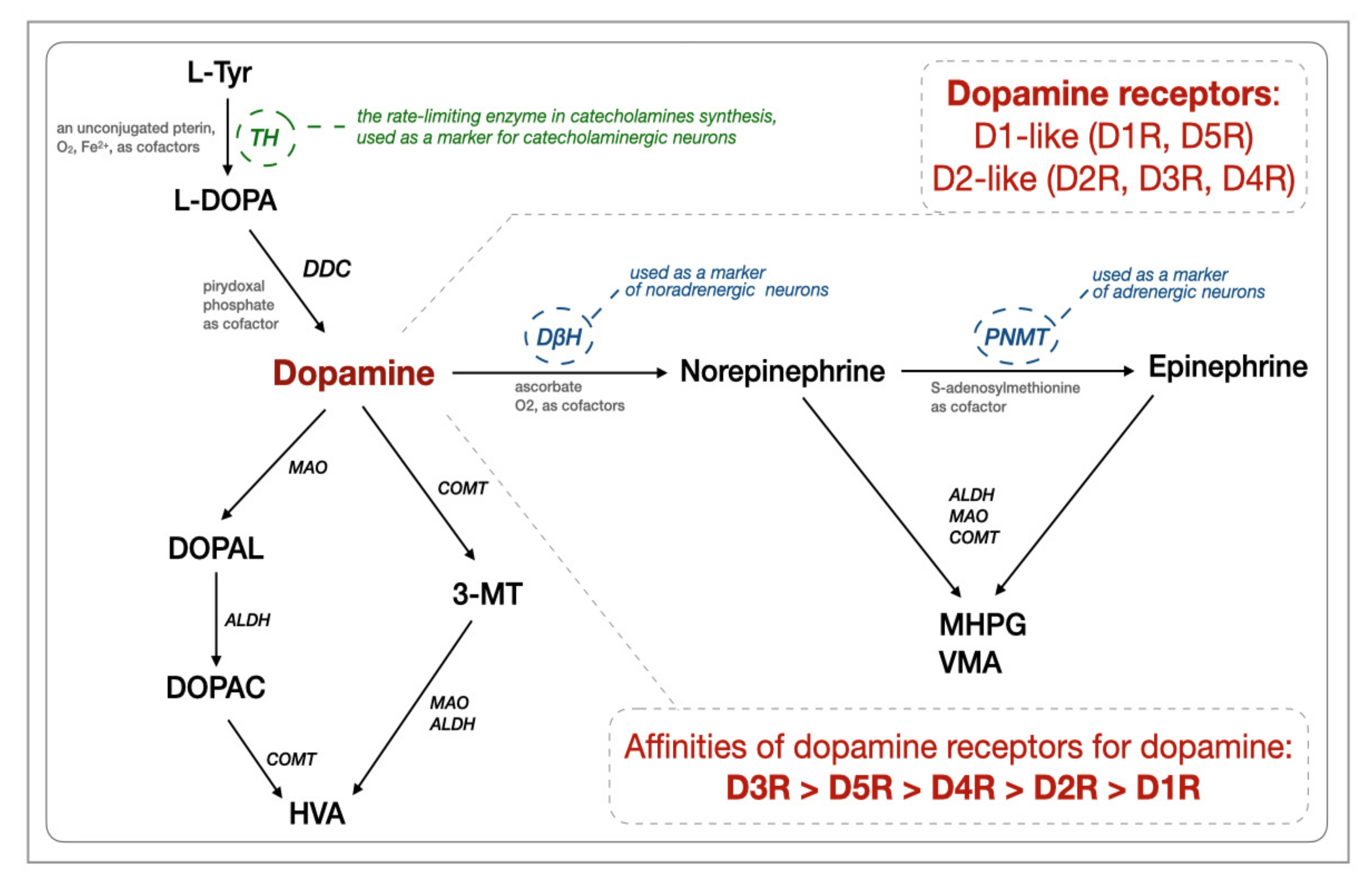This image presents a comprehensive, detailed diagram of the interaction and synthesis pathways of various neurotransmitters, with a particular emphasis on dopamine and its associated receptors. The white background, bordered by two grayish lines, frames the intricate connections between L-tyrosine (L-TYR), L-DOPA, dopamine, norepinephrine, and epinephrine. The diagram features multi-directional arrows illustrating the biochemical transformations: 

1. **L-tyrosine (L-TYR) to L-DOPA**: An arrow labeled 'TH' (the rate-limiting enzyme in catecholamines synthesis, marked in a green dashed circle) points downwards to L-DOPA, with an adjacent label 'PERIDOXAL PHOSPHATE as cofactor'.
2. **L-DOPA to Dopamine**: Another arrow labeled 'DDC' (DOPA Decarboxylase) directs from L-DOPA to dopamine. 
3. **Dopamine Pathways**: Dopamine is central, branching out in multiple directions:
   - **To Norepinephrine**: An arrow moves to norepinephrine, which is linked further to epinephrine.

Additional pathways involve enzymes MAO, ALDH, COMT facilitating the conversion of dopamine to DOPAL, DOPAC, HVA, and 3-MT.

In the upper right corner, the dopamine receptor types are categorized in red text: D1-like (D1R, D5R) and D2-like (D2R, D3R, D4R). The affinities of these receptors for dopamine are detailed at the bottom in a ranked list (in red): D3R > D5R > D4R > D2R > D1R.

Overall, this diagram not only maps out the metabolic pathways of these neurotransmitters but also highlights key regulatory enzymes and receptor affinities, encapsulating complex biochemical interactions in a visually structured format.